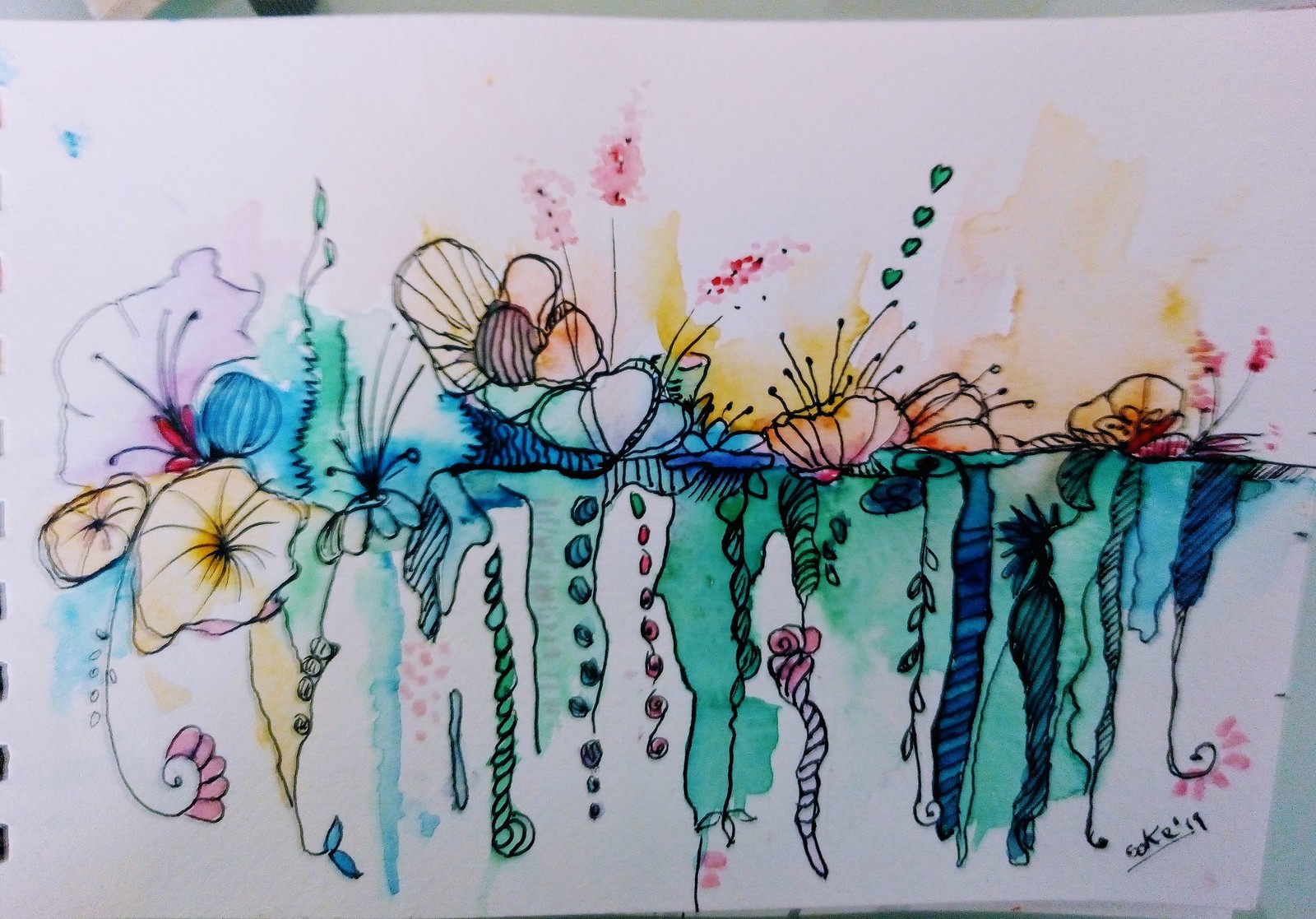This photograph showcases a detailed ink sketch of flowers, beautifully rendered in a combination of ink and watercolor. The floral design features distinct black lines that elegantly depict the flowers, petals, cascading buds, and stems, all set against a pristine white paper background. The watercolor fills the sketch messily yet artistically, spilling over the edges to create a captivating, artsy appearance. The vibrant colors—orange, yellow, and blue—add a stunning pop to the piece, enhancing its visual appeal. The artwork, which appears suitable even as a tattoo stencil, is signed in the bottom right corner with the letters "C or G-O-K-E,' 19," underlined for emphasis.